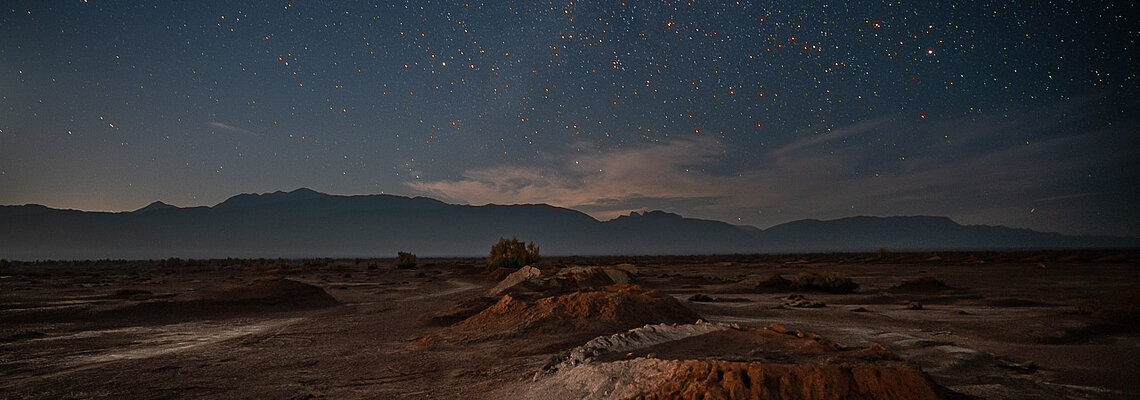This captivating photographic image captures an expansive, desolate landscape at night. The scene showcases a rugged foreground dominated by brown soil and rocky terrain, reminiscent of the edge of a crater. In the mid-ground, sparse trees are interspersed within the dusty, dry soil, adding a touch of vegetation to the otherwise barren environment. Stretching across the wide image in landscape mode, a series of gray, low-lying mountains forms the backdrop, their subtlety contrasting with the dramatic sky above.

The sky tells a vivid story of transition from day to night, with remnants of an orange sunset illuminating the clouds near the horizon. Above this fiery display, the sky deepens into darker shades of gray and blue, dotted with countless twinkling stars. The combination of the setting sun's glow and the emerging night sky creates a striking visual gradient. The photograph, devoid of any text or human presence, transports the viewer into a serene, almost otherworldly desert-like setting, perhaps inspired by the Midwest or a similar arid locale. It emphasizes the raw beauty and vastness of a remote, untouched landscape under a starlit sky.